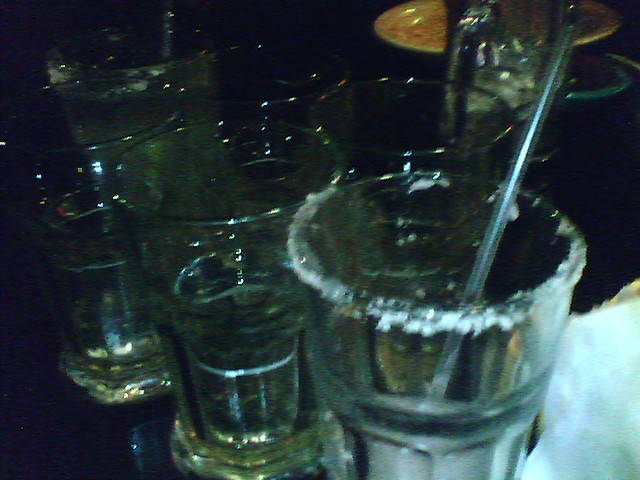In this dimly lit, blurred image likely taken at a bar, a table is cluttered with six mostly empty glasses. The glass closest to the camera has a clear straw sticking out and salt around its rim, indicating it likely contained a margarita. The other five glasses, suitable for serving beer, are empty and all are positioned in the foreground. Partially hidden behind the glasses in the upper right corner of the image is a dirty, light yellowish plate with remnants of what appears to be tomato sauce. The overall scene is dark, with very little detail visible in the blacked-out background, except for a partial glimpse of a person’s hand near the margarita glass.